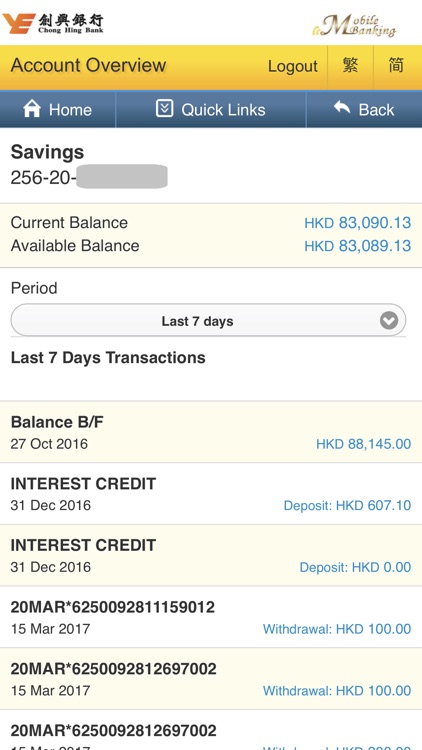This detailed screenshot showcases a banking interface, likely from a mobile app or website, prominently displaying the Y.E. logo accompanied by small, unreadable black Chinese lettering at the top left, possibly indicating "Ching Ming Bank" or "Ching Hing Bank." Below, a yellow bar or box appears, featuring an account overview section, a logout button, and two Chinese characters. 

Underneath this yellow section, a blue rectangular box labeled "Home" appears alongside categories including "Home" and "Quick Links," with a left-pointing arrow labeled "Back." Further down, the text "Savings" is seen in mixed-case typography, followed by the partially redacted account number "256-20-xxxx" in gray. The account details reveal a current balance of HKD 83,090.13 and an available balance of HKD 83,089.13 in Hong Kong Dollars.

The interface also shows a filters section to view transactions over various periods, with the last seven days selected. Below, it lists transactions from October 27, 2016, to April 15, 2017, detailing deposits and withdrawals with corresponding amounts displayed to the right.